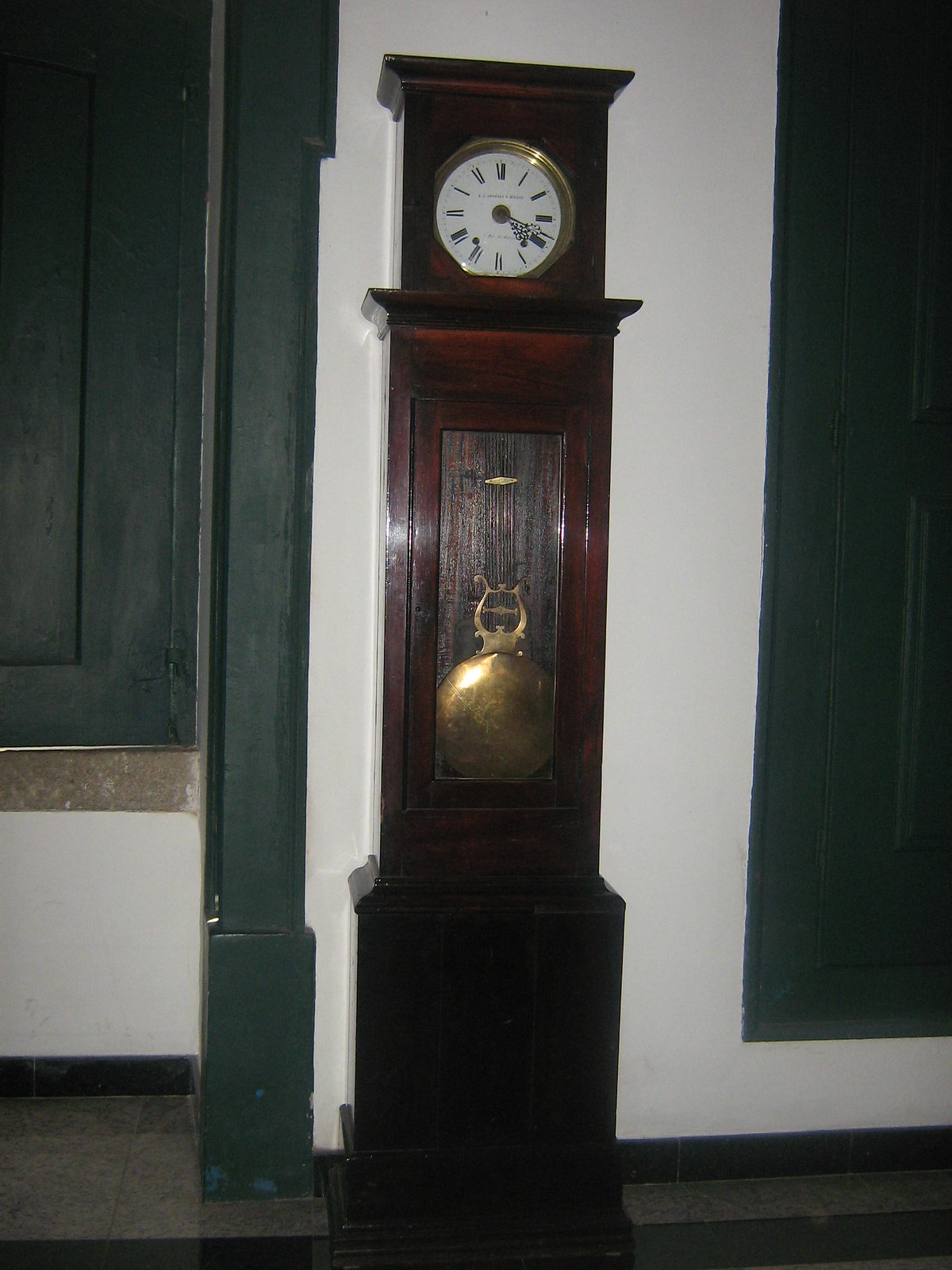A majestic grandfather clock stands regally against a pristine white wall. The clock, crafted from deep mahogany wood, exudes timeless elegance. Flanking this stately timepiece, door and window trims are painted a rich hunter green, providing a striking contrast. The centerpiece of the clock is its large, mesmerizing pendulum, visible through a glass window in the center. At the summit of this towering structure, a brass-framed clock face gleams, displaying black Roman numerals on a pristine white background. The ornate hour and minute hands, also fashioned from brass, add an extra touch of sophistication. The base of the cabinet is simple yet refined, maintaining the deep mahogany hue. Below, the floors are a stunning display of gray and black marble, further enhancing the clock’s distinguished presence in the room.